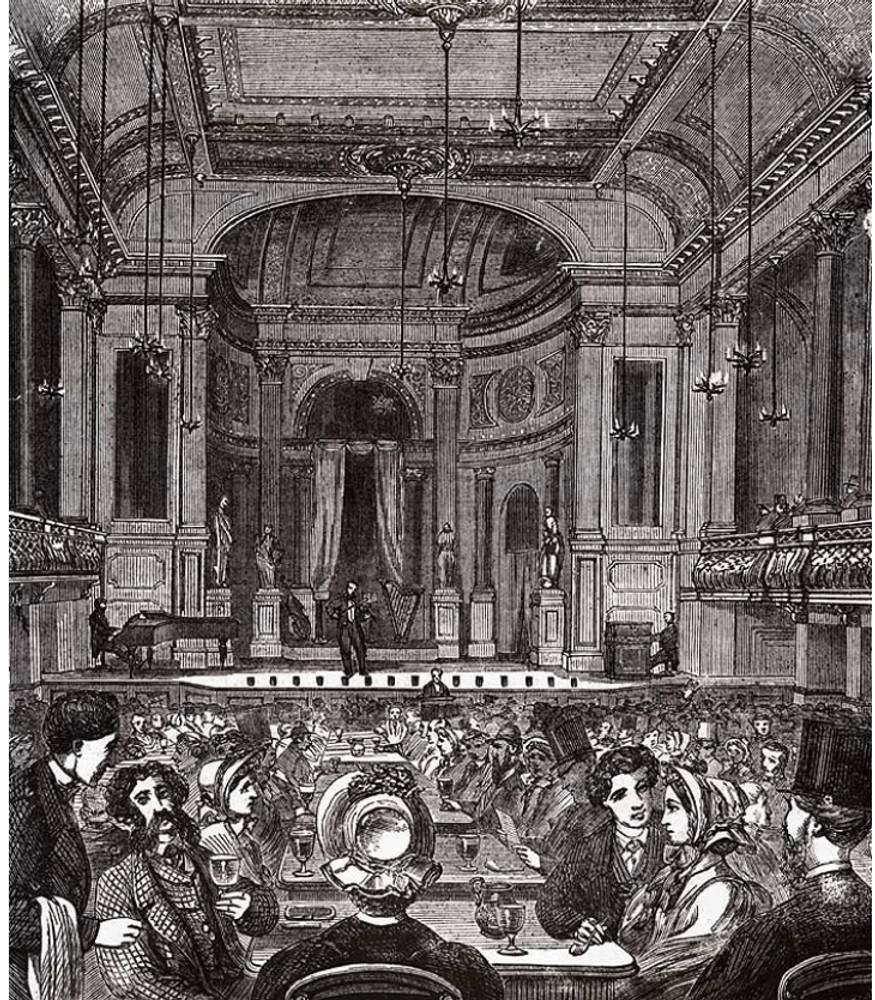This detailed black-and-white drawing, tinted with shades of brown, captures an elaborate and highly detailed scene inside a large, ornately decorated room. The room, featuring a tall, curved ceiling with candle chandeliers hanging from long strings, evokes an atmosphere of historical grandeur. At the heart of the image is a stage with a tall archway adorned with pillars and statues. Onstage, a man centrally positioned plays a violin, with fellow musicians accompanying him on a grand piano to the left and possibly an organ to the right. This performance unfolds before an audience seated at numerous tables, where they socialize, drink wine, and enjoy the music. The elegantly dressed attendees, in top hats, dresses, and suits, fill the lower portion of the image. Notable details include a waiter attending to a man holding a wine glass on the lower left, and at the head of one table, a figure assumed to be a woman with a flowered bonnet. The intricate detailing of the room and its occupants suggests an old etching or print of a lavish banquet or orchestra hall.